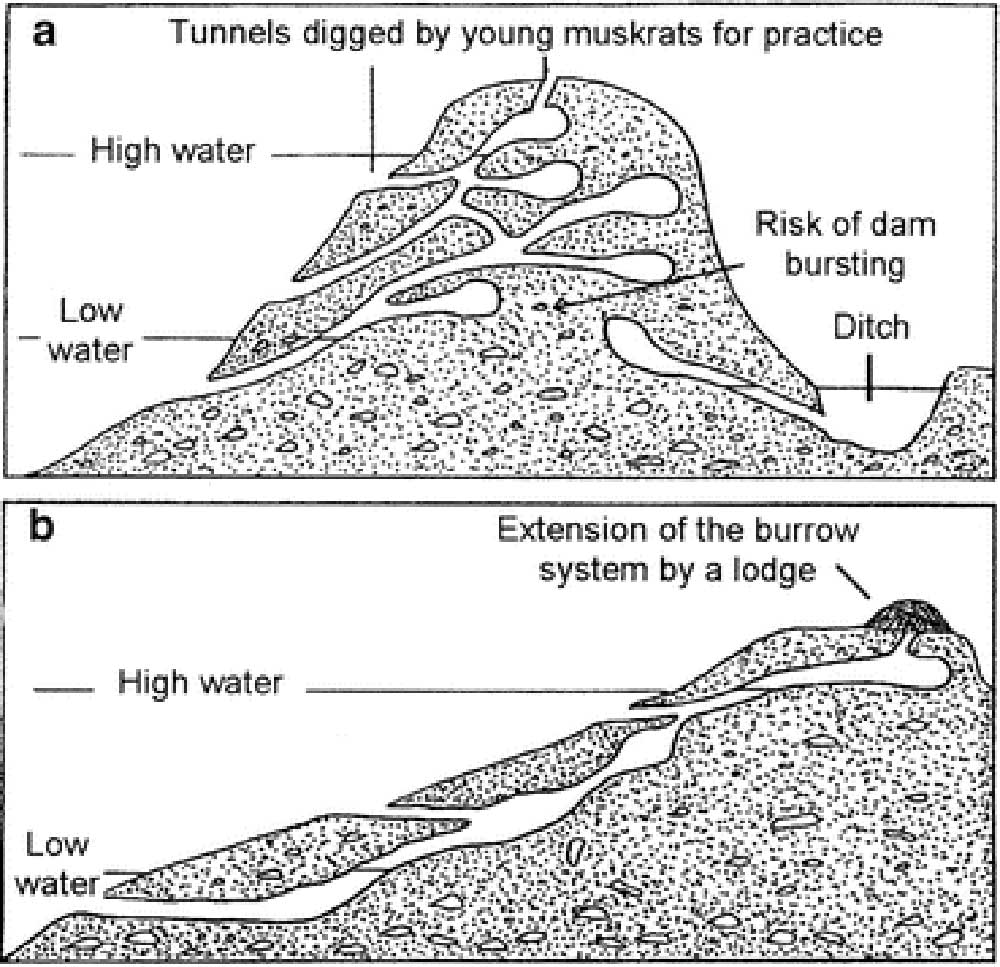The image features two black-and-white diagrams labeled A and B, resembling illustrations from a textbook. Diagram A, occupying the top half, provides a cross-sectional view of a hill, with various tunnels excavated by young muskrats for practice. Labels denote significant features such as "high water," "low water," "risk of dam bursting," and a "ditch." Diagram B, placed below, displays an extension of the burrow system leading to a muskrat lodge situated atop a hill. Similar to the first diagram, it indicates high and low water marks and illustrates a network of tunnels connecting the body of water to the lodge, providing detailed insights into muskrat habitat and behavior.